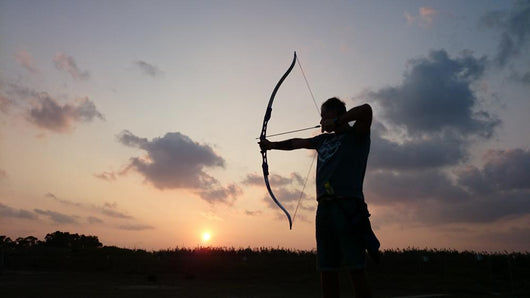This photograph, taken either at sunrise or sunset, beautifully captures the serene moment of a man engaging in archery. The scene is set against a stunning sky that transitions from a golden peach hue near the horizon to a deeper, dusky blue towards the top. Puffy, dark grey clouds and cirrus clouds are scattered across the sky, adding texture to the peaceful backdrop. The man, standing slightly off-center to the right of the image, is silhouetted against this dramatic sky, making it difficult to discern details of his appearance, though he appears to be wearing a t-shirt and possibly has short hair.

The photograph is taken from a lower perspective, making the man appear even more imposing as he stands tall with his bow and arrow. His right hand is drawn back, ready to release the arrow, while his left hand keeps the bow steady, aiming towards the left side of the frame. In the background, you can see the sun—a distant golden glow low on the horizon—partially obscured by silhouettes of trees and tall grasses or bushes. The overall scene exudes a sense of calm and focus, perfectly capturing the stillness of the moment before the arrow is released.